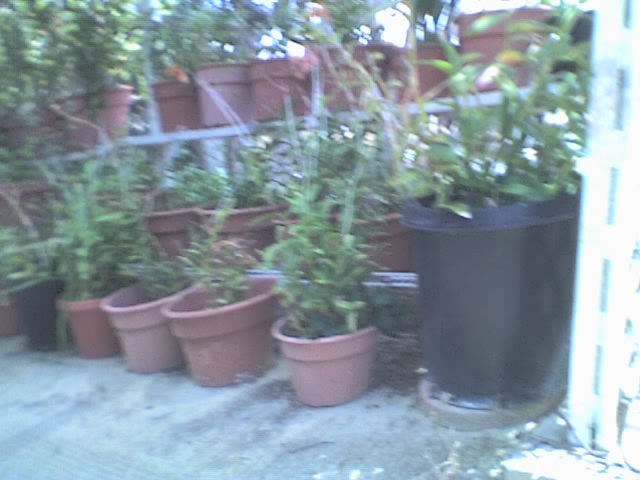This image features an assortment of potted plants arranged neatly on a light gray concrete floor under bright sunlight streaming from the top right corner. The focal point of the arrangement is a combination of reddish-orange clay pots and dark black pots. The largest of the pots, a dark black one, houses a lush green vine that cascades elegantly out of it. To its right, another black pot at the end of the first row holds a similar verdant fern-like plant. Among the variety of plants, all feature green leaves in various shapes and sizes, with some plants having leaves that slightly extend past the rims of their pots, but none of the plants are flowering.

This curated garden is organized meticulously in a tiered metal rack that resembles a wooden trellis, containing three rows of pots, each row slightly higher than the one in front. The structural frame of the pot holder stands out with its white bars, creating a gentle contrast against the colorful pots and greenery. The overall composition, with its healthy green plants and strategic lighting, suggests a serene and well-maintained plant display, possibly situated in a green corner of a store or garden center.